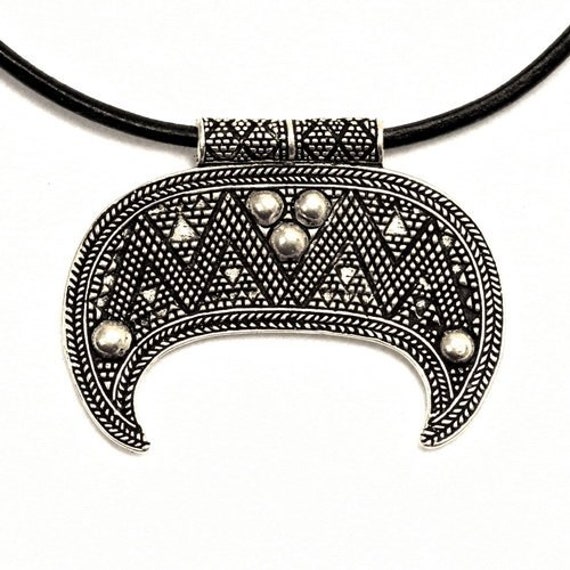The image showcases a detailed close-up of a choker-style necklace, with the focus on its intricate pendant. This necklace features a black, wiry cable that likely wraps around the wearer's neck. The pendant, shaped like a downward-facing half-moon crescent, predominantly displays a silver color with various patterns and details.

The crescent moon pendant is adorned with black embedded zigzag lines, forming what appears to be two interconnected M shapes. Along the trim of this crescent, several small, silver, ball-like decorations are positioned: one on the left, one on the right, and three clustered together in the center. Additionally, the pendant surface includes small, silver, triangular spots that enhance the geometrical appeal of the design. The pendant is attached to the choker by a cylindrical loop, through which the black cable runs, ensuring it hangs securely. The overall appearance of this trendy accessory is reminiscent of fashion items one might find at a store like Claire's, adding a stylish, modern touch to any outfit. The shadow of the pendant is visible below it, indicating a well-lit and slightly elevated photographic angle.